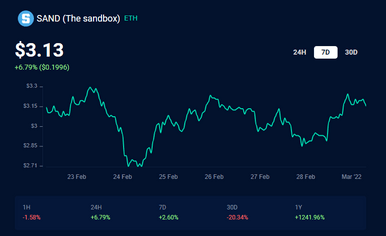A small, somewhat blurry screenshot, likely from the Robin Hood app, features a dark, almost black or deep blue background. At the top of the image, the word "sand" is prominently displayed, accompanied by the term "dust sandbox" in parentheses. The screenshot shows a financial graph with both red and green indicators, illustrating trends over several months. The graph includes a green upward trend line, juxtaposed with red negative markers, suggesting fluctuations in value. In the lower part of the image, a monetary figure is visible, reading three dollars and thirteen cents ($3.13).